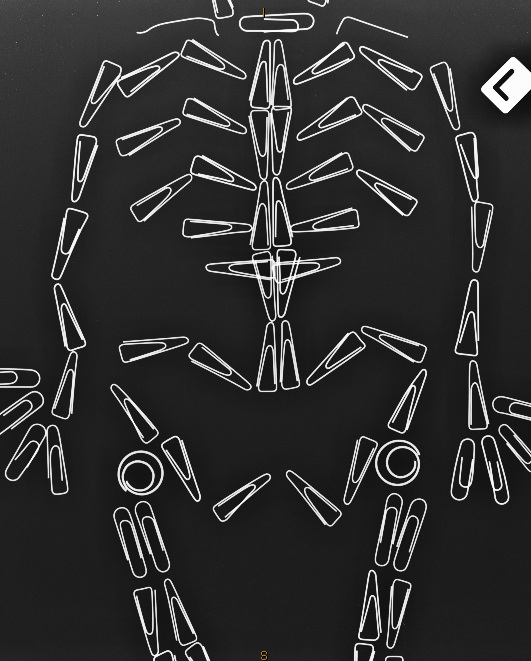Against a stark black backdrop, a meticulously arranged collection of white paperclips forms an intricate and detailed human skeleton. This artistic creation employs a variety of paperclip shapes, including familiar rounded clips, triangular clips reminiscent of candy corn, capsule-shaped, and circular ones. These diverse paperclips are expertly positioned to depict the skeletal structure with remarkable accuracy. The arrangement outlines the clavicle, spine, ribcage, arms with fingers, pelvis, and legs down to the femur. Adding a touch of authenticity, a white rectangle with the letter "L," akin to a traditional x-ray marker, tilts at an angle in the top right corner of the image. This captivating piece might be a computer-generated art, capturing the skeletal form in a striking black-and-white color scheme, highlighted by the contrast between the white paperclips and the dark background.